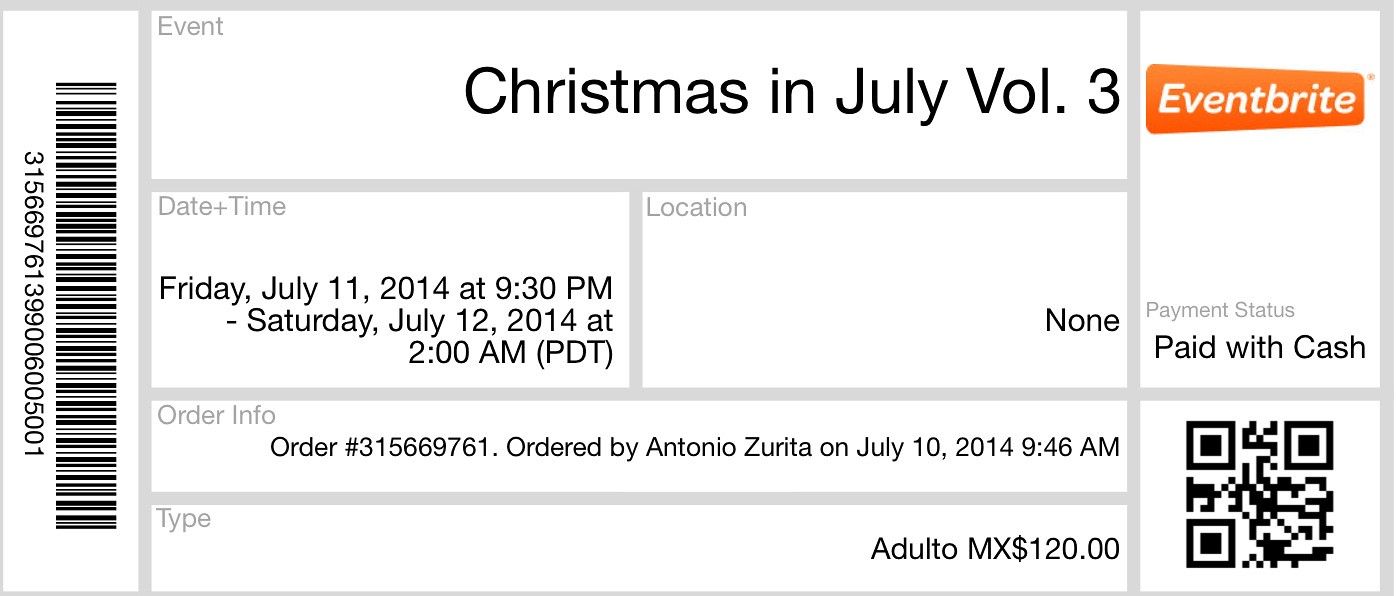The image showcases an Eventbrite ticket, presented in a white, horizontal format, meaning it is wider than it is tall. The Eventbrite logo is prominently displayed in the top right-hand corner, featuring a rounded orange rectangle with the word "Eventbrite" in white. Across the top line in bold text, the event name is "Christmas in July Volume 3." Beneath the event name in the top panel, various details are listed: 

- **Date Time:** Friday, July 11, 2014, at 9:30 p.m. and Saturday, July 12, 2014, at 2:00 a.m. PDT.
- **Location:** None.
- **Order Information:** Order Number 315-669-761, ordered by Antonio Zurita on July 10, 2014, at 9:46 a.m.
- **Type:** Adulto MX $120.
- **Payment Status:** Paid with Cash.

The ticket also includes a QR code located in the bottom right-hand corner and a barcode on the left-hand side with the number "315-669-761-399-006-005-001" underneath it. The overall design is a monochromatic print publication with spot color in orange, giving it a clean and professional appearance.